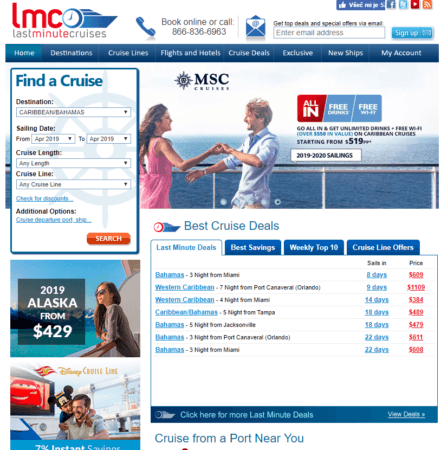The screen capture from the "Last Minute Cruises" website prominently features the logo LMC alongside a clock face and a cruise ship, symbolizing prompt and immediate cruise deals. The header includes a booking prompt encouraging users to either "Book Online" or call a provided phone number. The central image depicts two people standing at a railing, likely on a cruise ship, enjoying their aquatic adventure.

The website offers interactive search options with criteria such as "Find a Cruise," "Sailing Date," "Cruise Length," "Cruise Line," and "Additional Options," accompanied by a "Search" button. A highlighted promotion mentions "2019 Alaska from $429," although it’s unclear if this rate is per person or per night, necessitating a click for more details.

Additional sections featured on the site include "Last Minute Deals," "Best Savings," "Weekly Top Ten," and "Cruise Line Offers." These sections likely aim to fill vacant rooms at discounted rates, ensuring fully booked cruises by offering significant savings to last-minute travelers.